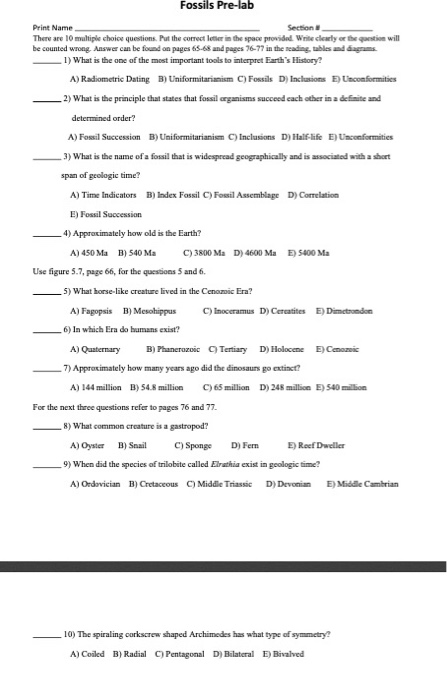This is a detailed screenshot of a test or quiz titled "Fossils Pre-Lab" at the top. Directly below the title, there are two fields for filling out information: one for "Print Name" which is followed by a large underline to its right, and another for "Section Number," also with a large underline to its right. 

Below these fields, there is a paragraph in serif black text giving instructions for the quiz. The paragraph reads: 

"There are 10 multiple choice questions. Put the correct letter in the space provided. Write clearly or the question will be counted wrong. The answer can be found on page 65 to 68 and pages 66, 76 through 77 in the reading tables and diagrams."

Following these instructions, the multiple-choice questions are listed vertically. Each question has a designated line to the left of its number for entering the answer. To the right of each number, the corresponding question is displayed, followed by the answer choices arranged under it. The first four questions are as follows:

1. What is one of the most important tools to interpret Earth's history?
   - A. Radiometric dating
   - B. Uniformitarianism
   - C. Fossils
   - D. Inclusions
   - E. Unconformities

2. What is the principle that states that fossil organisms succeed each other in a definite and determined order?
   - A. Fossil succession
   - B. Uniformitarianism
   - C. Inclusions
   - D. Half-life
   - E. Unconformities

3. What is the name of a fossil that is widespread geographically and is associated with a short span of geologic time?
   - A. Time indicators
   - B. Index fossils
   - C. Fossil assemblage
   - D. Correlation
   - E. Fossil succession

4. Approximately how old is the Earth?
   - A. 450 million years old
   - B. 540 million years old
   - C. 3,800 million years old
   - D. 4,600 million years old
   - E. 5,400 million years old